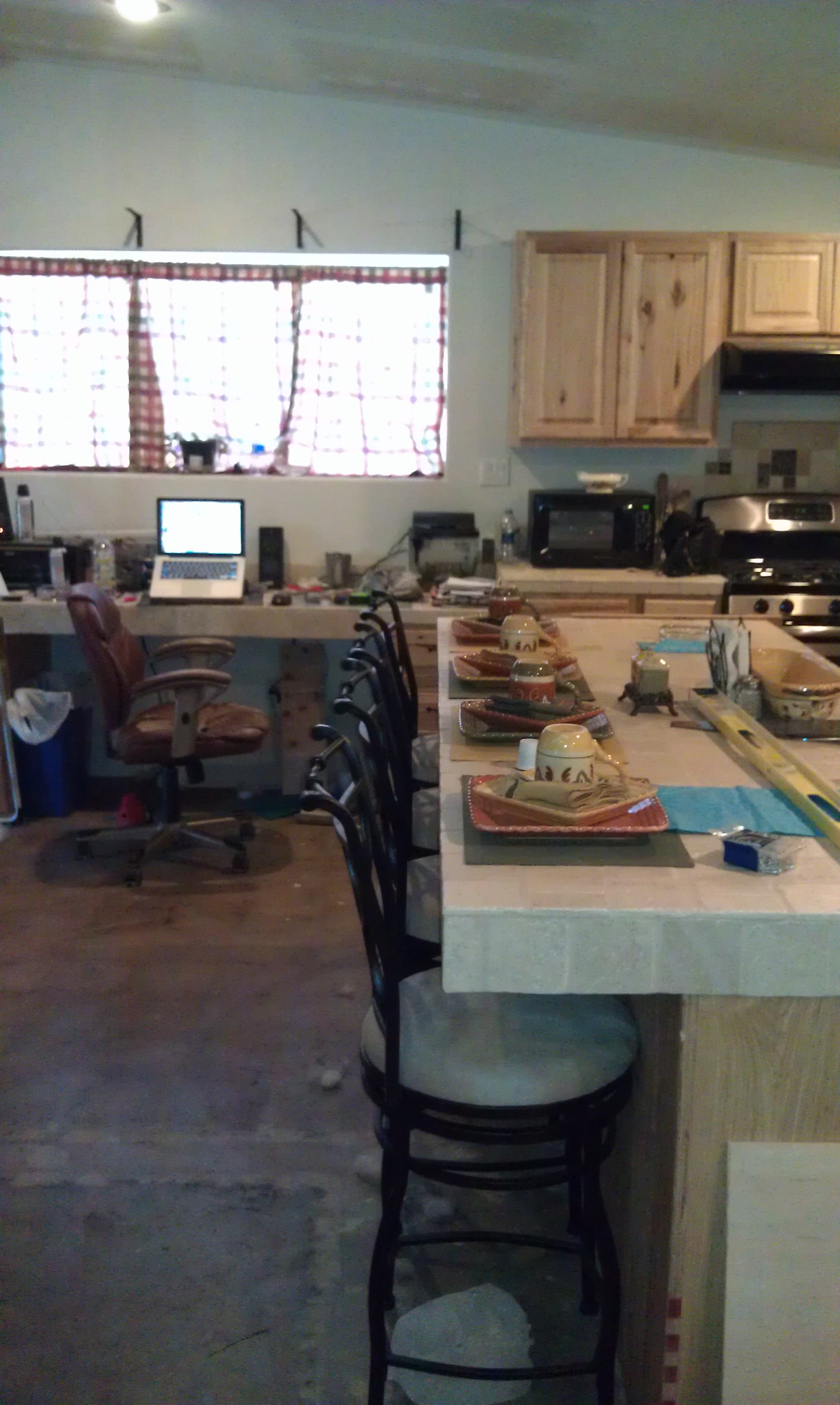This photograph captures a diverse living space combining a kitchen, dining area, and office within a large, segmented room. In the top right corner, against an off-white wall, there are beautiful natural wood finish cabinets mounted on the wall. Below these cabinets, a sleek black and silver stove and a microwave seamlessly blend into the cabinetry. Directly beneath the microwave, additional cabinets of the same wood finish provide cohesive storage.

On the bottom right, extending along the right side, a butcher block dining table stands out with its thick natural wood surface. Arranged along the left side of this table are four elegant chairs, each featuring black frames and white seats. Each place setting is meticulously prepared for dining. Unusually, a long yellow level stretches across the center of the dining table despite it being formally set for dinner.

On the left-hand top side of the image, a trio of connected windows is adorned with thin red and white checkered curtains, allowing a view through them. Below this window arrangement, a countertop matching the dining table’s butcher block style transitions into an office space. This area is organized yet occupied with daily essentials, including a printer on the far left, a laptop tilted on a stand in the center, and a speaker accompanied by various gadgets and clutter on the right. A brown leather office chair on wheels is positioned in front of the laptop, complementing the workspace ambiance. Lastly, a royal blue trash can with a white liner nests underneath the left corner of the table, maintaining convenience at arm's reach.